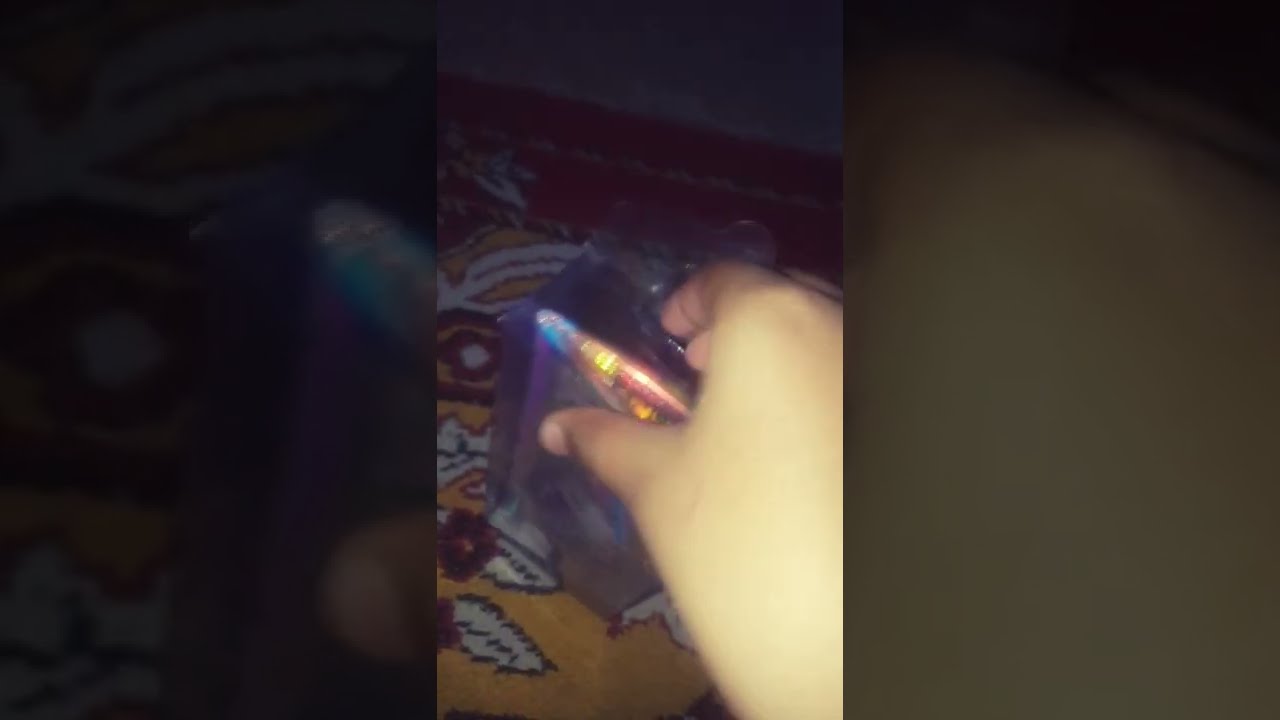The image is a vertically-oriented cell phone photograph featuring the right hand of what appears to be a young person. The hand is reaching forward from the bottom right edge, gripping a semi-transparent plastic case. Inside the case, a glossy pink vial with a gold top and other partially visible items can be seen, suggesting that it might be a makeup kit. The hand and the object are centered in the photograph, which has a background made up of a zoomed-in, darkened, and faded portion of the same image on both the left and right. The object rests on a vibrant surface that appears to be a fabric with a geometric and floral pattern in hues of gold, orange, red, and white. The photograph is dark and somewhat blurry, adding to its realistic yet slightly obscured feel.